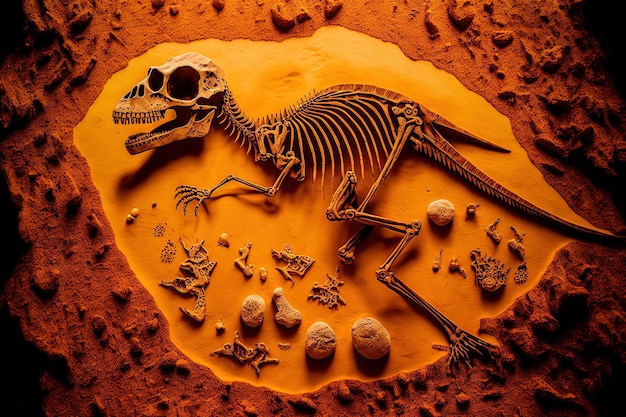The image depicts a nearly complete skeleton of a bipedal dinosaur, likely a Tyrannosaurus Rex, arranged as though it is encased in amber or a similar substance. This skeleton is positioned in the center of the image, with its head pointing to the left and its long tail extending to the right. The dinosaur has long back legs and shorter front legs, and it appears to be lying on the ground. The background immediately surrounding the skeleton is a bright yellow-orange, resembling amber, which transitions to a rocky orange texture, and eventually fades into black at the corners of the image.

The dinosaur skeleton is surrounded by various other fossilized objects, including some that resemble invertebrates and possibly fossilized eggs, with at least three egg-like shapes visible—two near the back legs and one near the right hand. The fossilized remains and assorted bones are embedded within the yellow area, giving the impression of an archaeological discovery. The yellow-orange background casting shadows hints at sunlight filtering through, enhancing the three-dimensional appearance of the scene. Overall, the intricate details make the image reminiscent of a prehistoric preservation similar to the iconic Jurassic Park logo.